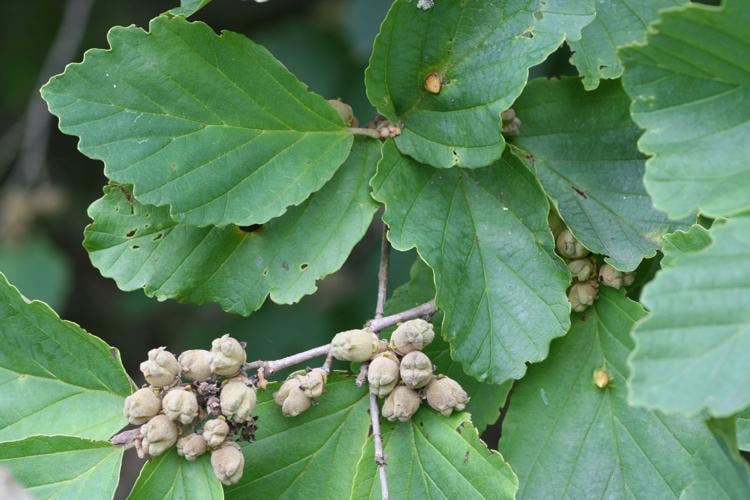This is a detailed close-up color photo of a tree or plant, featuring vibrant green leaves that dominate the image, making the background a blurred, indistinct presence. The leaves, some of which exhibit small holes likely caused by hungry insects, have scalloped edges and are arranged in various directions. Prominently interspersed among these leaves are clusters of small, round, brownish-white seeds or nuts. These seeds, which resemble acorns or closed balls, often display a cross-like structure at their ends, akin to the head of a screw. Some of the leaves also show sharp, thorny protuberances, adding to the texture of the scene. The focus on the green leaves and the detailed seeds gives the photo a rich, immersive quality, capturing the intricate beauty and minor imperfections of nature.